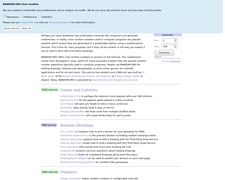The image features a blue rectangle, approximately four inches in length, containing various lines of text that are extremely blurry and unreadable. The first line of text is in a darker black font. Directly beneath this, additional lines of information are present, rendered in slightly lighter text. Proceeding down the rectangle, there is a white rectangle with small black text inside, followed by a paragraph that is entirely illegible due to its very small lettering. This paragraph is also in black text, and another similarly unreadable paragraph follows below it.

To the left side of the image, a subheading appears in green text, but it is far too small to decipher. Adjacent to this subheading on the right, there are pieces of information presented in both light blue and black text. Below this section, dark blue words are visible, followed by approximately eight lines of text. These lines alternate between light blue and black colors. The image concludes with medium green text, small light black text next to it, and finally, darker black text.